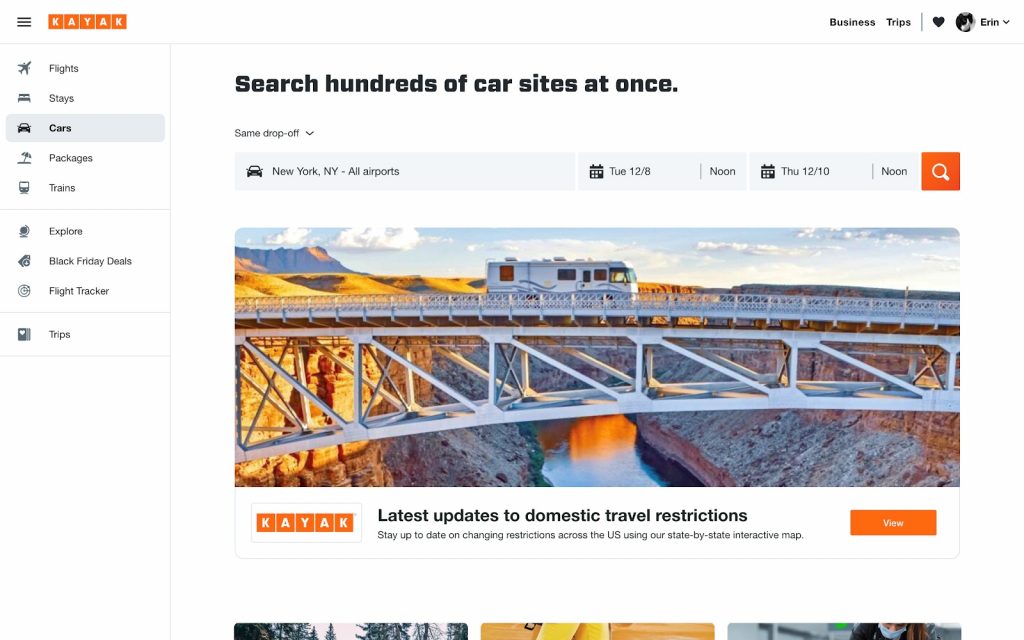In the image, the interface of a travel booking platform is presented with various elements clearly laid out. 

At the top-left corner, the word "kayak" is prominently displayed in white text on an orange square-patterned background. Adjacent to this is a black hamburger menu icon, consisting of three horizontal bars. Also in the upper left, the username "grin" is visible beside a heart symbol, along with the words "trips" and "business".

Underneath these elements, there is a row of categorized options including "flights," "stays," "cars," "packages," and "trains." The "cars" category is currently highlighted with a distinctive greenish-blue background. Below this row, additional options such as "explore," "Black Friday deals," and "flight tracker" are listed.

Dominating the center of the image is a search area labeled "Search hundreds of cars, sites at once." Below this heading, several input boxes are arrayed. The first box, positioned on the far left, reads "New York, New York, all airports." To the right of this, date selection boxes are displayed, with the first box indicating "Tuesday 12-8" and the second box showing "Thursday 12-10."

At the bottom of the image, a large rectangular photo captures attention: it depicts a scenic bridge with an RV driving across it, enhancing the travel-oriented theme of the platform.